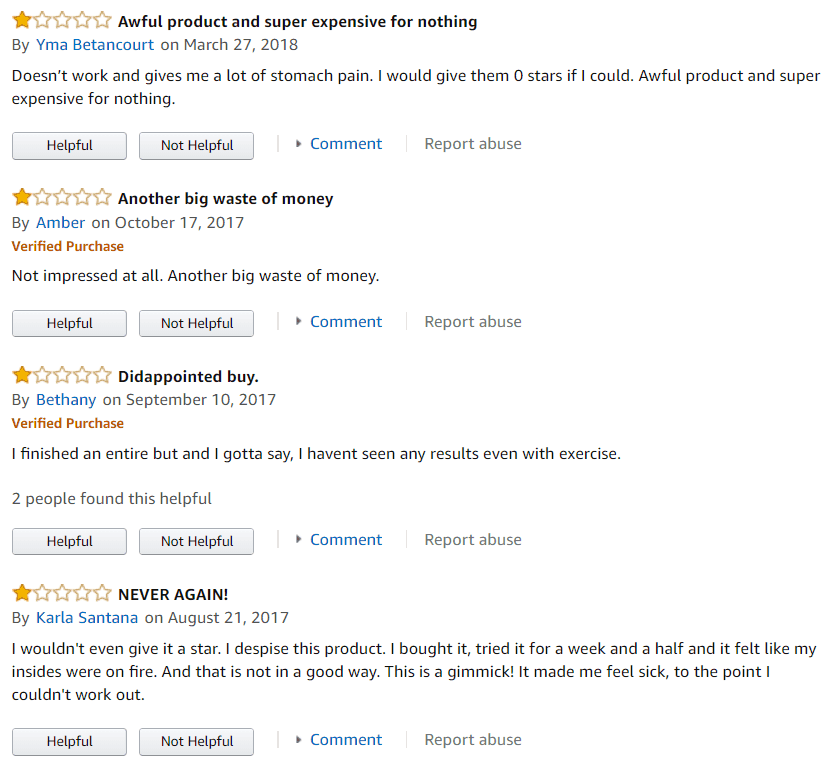**Descriptive Caption:**

The image depicts a sharply vertical, rectangular screenshot resembling an Amazon review page filled with negative feedback. Each review is formatted with a 4-star rating system where only the first star is gold, indicating a 1-star rating. Here’s a detailed breakdown of the reviews from top to bottom:

1. **Review by YMA Bentecourt (March 27, 2018):**
   - **Title:** "Awful product and super expensive for nothing."
   - **Content:** "Doesn't work and gives me a lot of stomach pain. I would give them zero stars if I could. Awful products and super expensive for nothing."
   - **Interactive Options:** Below the review text are clickable gray boxes with "Helpful" and "Not Helpful" in black text, followed by a faint gray bar with a gray arrow pointing to the right, labeled "Comment" in blue, and another faint gray bar labeled "Report Abuse" in gray.

2. **Review by Amber (October 17, 2017):**
   - **Title:** "Another big waste of money."
   - **Content (Black text):** "Not impressed at all, another big waste of money."
   - **Additional Info:** Verified Purchase (in orange text). The same interactive options as the first review follow.

3. **Review by Bethany (September 10, 2017):**
   - **Title:** "Disappointed."
   - **Content:** "I finished an entire bottle, but I have to say I haven't seen any results even with exercise."
   - **Additional Info:** Verified Purchase (in orange text), and "Two people found this helpful" (in gray text). The same interactive options as the previous reviews follow.

4. **Review by Carla Santana (August 21, 2017):**
   - **Title (All caps with an exclamation point):** "NEVER AGAIN."
   - **Content:** "I wouldn't even give it a star. I despise this product. I bought it, tried it for a week and a half, and it felt like my insides were on fire, and not in a good way. This is a gimmick. It made me feel sick to the point I couldn't work out."
   - **Interactive Options:** The same as the other reviews.

**General Observation:**
The reviews likely pertain to a weight loss or exercise product, and unanimously reflect negative experiences. Each comment warns of the product’s ineffectiveness and adverse effects, contributing to a consensus that the product is not worth trying.